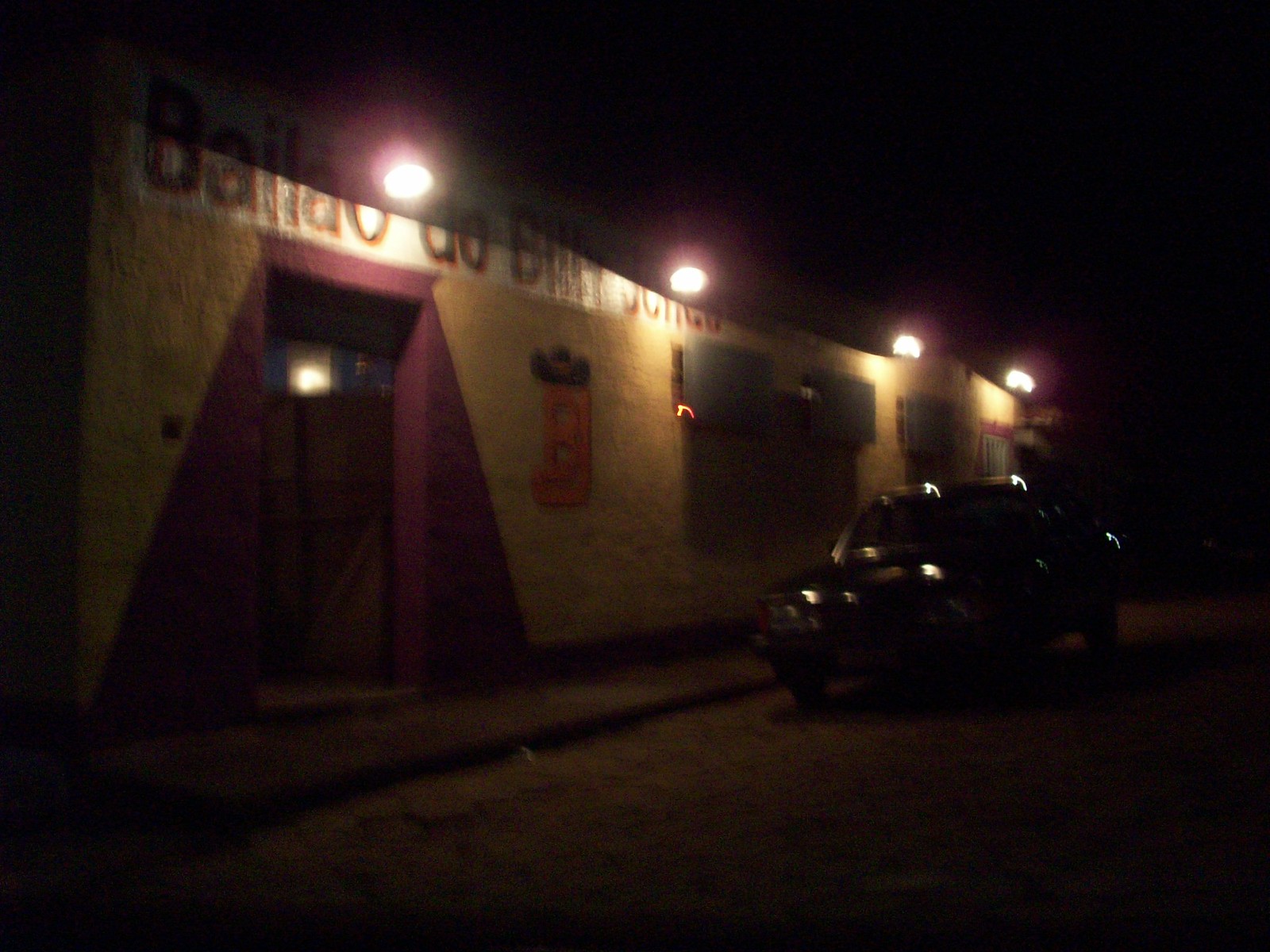In this nighttime setting, an image captures a building prominently featuring Western saloon-style doors in the center, painted yellow with distinctive triangle shapes around the door and a rectangular purple strip overhead. Illuminated by four lights, the facade includes windows with awnings and a sign displaying the word "by Lau do Billy" in a foreign script, beneath a logo of a "B" and "J" adorned with a cowboy hat. To the bottom right, a black car is parked along a roadway next to a curb, adjacent to a narrow sidewalk. The overall scene, appearing somewhat blurred, suggests the building may be a bar or restaurant surrounded by a mix of dark hues and vibrant tones like black, white, tan, maroon, orange, and green.